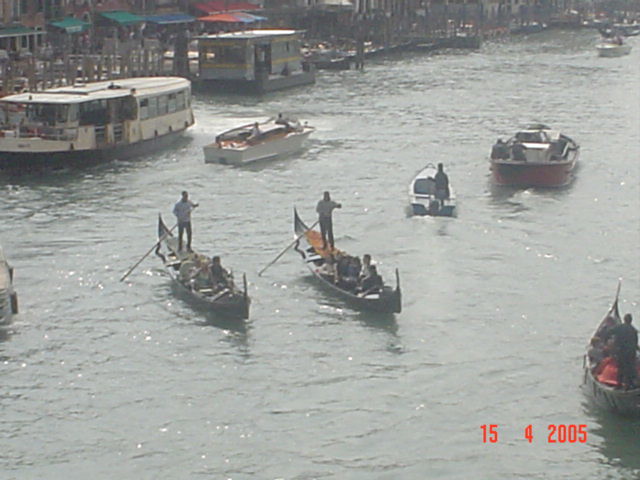This photograph, dated April 15, 2005, shows a vibrant river scene with a washed-out color palette, suggesting either early morning or late evening lighting. The river, wide and bustling with activity, features several types of boats. Prominently, there are two traditional gondola-shaped boats, each manned by a person standing at the back with a long pole, navigating diagonally from the top left toward the bottom right of the image. Another similar gondola is situated in the bottom right corner. There are also multiple motorized fishing boats, some moving away from the camera and others scattered across the river.

On the left side of the river, the shoreline is lined with continuous low buildings adorned with awnings, creating the impression of a busy dock area. Wooden pilings support the waterfront structures, and houseboats, which appear worn and modest, are moored along the edge. A wooden structure with vertical beams and cloth canopy covers suggests a boardwalk bustling with activity, possibly market stalls or eateries. Behind this arrangement, larger houseboat-type vessels are also visible, contributing to the intricate and lively riverside atmosphere.